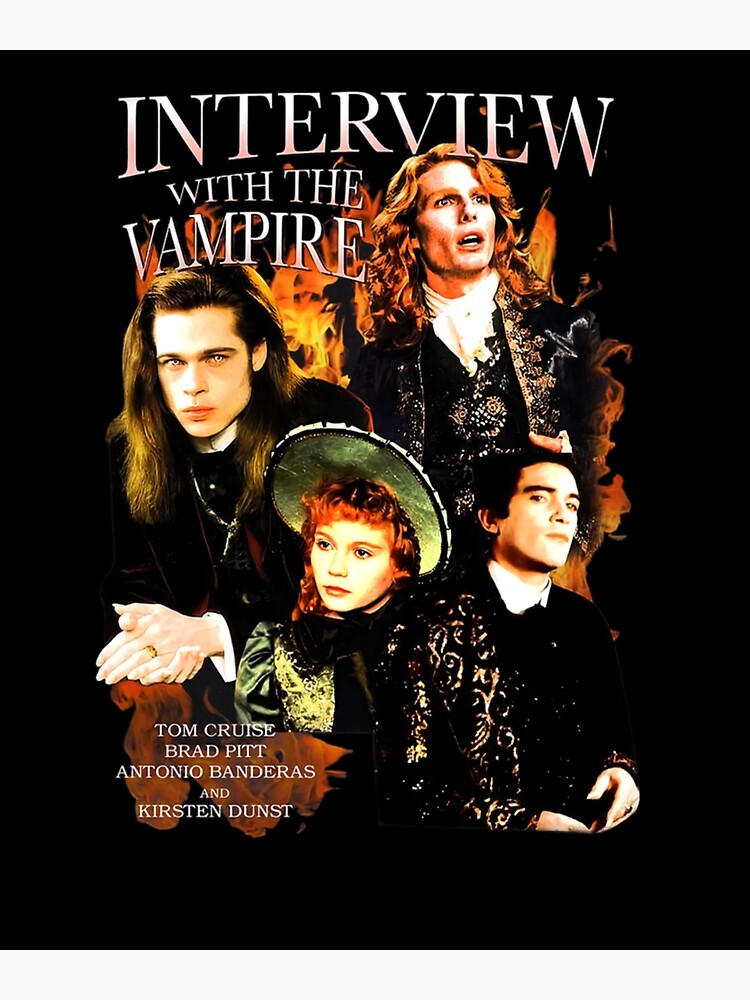The movie poster for "Interview with a Vampire" features a striking black background with the title prominently displayed at the top in bold, white-pink gradient letters. Below the title, the credits are listed in the lower corners, showcasing the names of the prominent cast: Tom Cruise, Brad Pitt, Antonio Banderas, and Kirsten Dunst.

In the center of the poster, amidst a backdrop of blazing flames, four characters are vividly portrayed. On the left, a young man with long blonde hair stares ahead with piercing blue eyes. To the right, another man with a layered cut of light blonde hair gazes slightly upward, exuding a mysterious allure. Dominating the top right under the title, a man with long red hair and a fanciful jacket adorned with a white collar stands out as the focal point of the image. In front of the three men, a young woman with curly red hair, donning a green ornate dress and a matching bonnet-style hat, completes the foreground. The arrangement and their intense expressions convey a captivating and dramatic aura, perfectly setting the tone for the film.